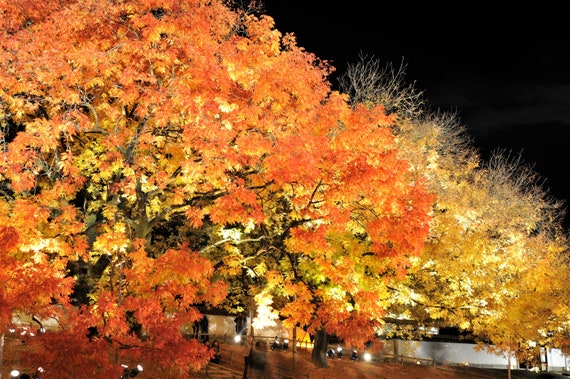This captivating nighttime photograph showcases a stunning display of several large, brightly colored trees with expansive branches. The foliage transitions from vivid orange on the prominent tree to the left, to an array of bright and golden yellows on the trees to the right, enhanced by illuminated spotlights from the ground. The leaves are extraordinarily vibrant, enveloping roughly 85% of the image with their luminous colors, while the top right corner reveals a stark contrast with the solid black night sky. The thick trunks of the trees stand tall above what appears to be a grassy field. Upon closer observation, two people can be seen sitting on the grass, possibly admiring the breathtaking view. In the background, a faint outline of a building suggests this scene might be set in a park. Although there are some leafless twigs at the top, the trees are mostly in full bloom, their radiant leaves highlighted by the strategically placed lights beneath them.